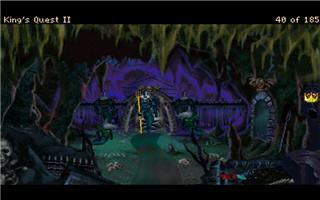This color screenshot is from the classic video game King's Quest II, showcasing its vintage, pixelated graphics. The scene is set in an eerie underwater cave adorned with numerous green, mossy stalactites that hang menacingly from the ceiling. The cavern floor is littered with human skulls and scattered bones, adding to the ominous atmosphere. In the background, an imposing throne is occupied by a menacing, fish-like creature clutching a trident, reinforcing the scene's dark and mysterious vibe. The top left corner of the image is labeled with "King's Quest II," while the top right corner indicates a game progress marker, "40 of 185." No text, buildings, or motorized vehicles are present in this detailed and atmospheric video game screenshot.